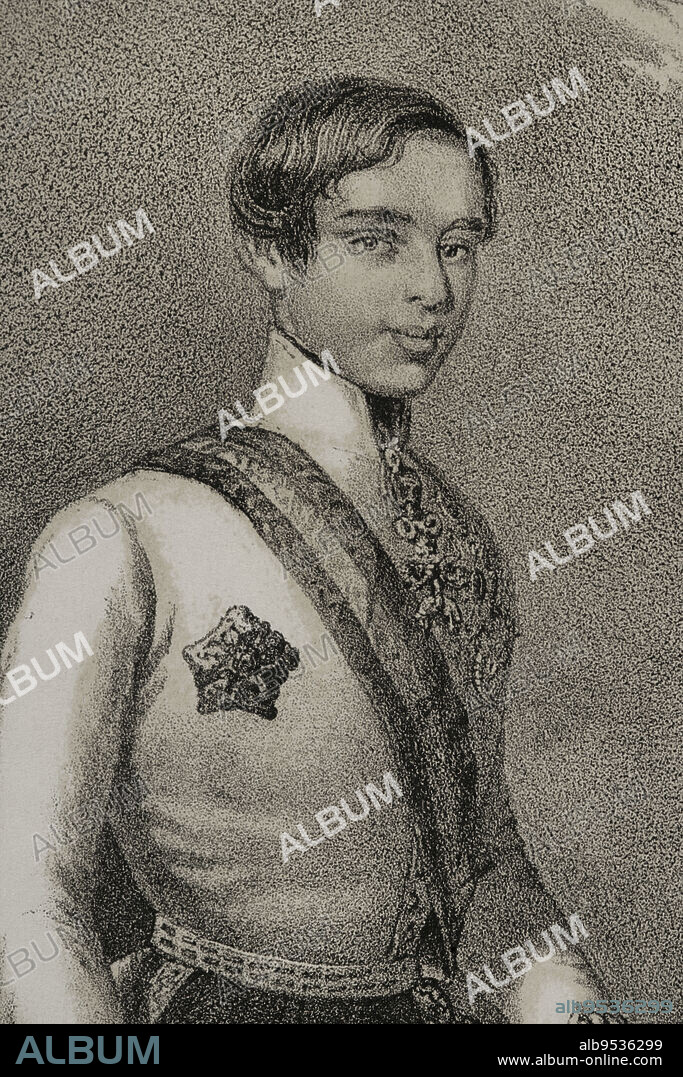The image is a vertically aligned rectangular black and white drawing of a young man, likely in his late teens or early twenties, dressed in an old-fashioned military uniform. His short hair is combed to the side with a slight curl, and his lips are together in a faint smile. He wears a sash diagonally across his right shoulder to his left waist, with a star-like badge pinned to his right chest, suggesting some military rank. The drawing, which appears to be vintage, possibly from the 1800s or 1900s, is watermarked repeatedly with the word "ALBUM" in white, printed diagonally across the image. At the bottom of the narrow rectangle is a black border where "ALBUM" is written in all caps green on the lower left. On the lower right, the code "ALB9536299" is displayed, followed by "www.album-online.com."